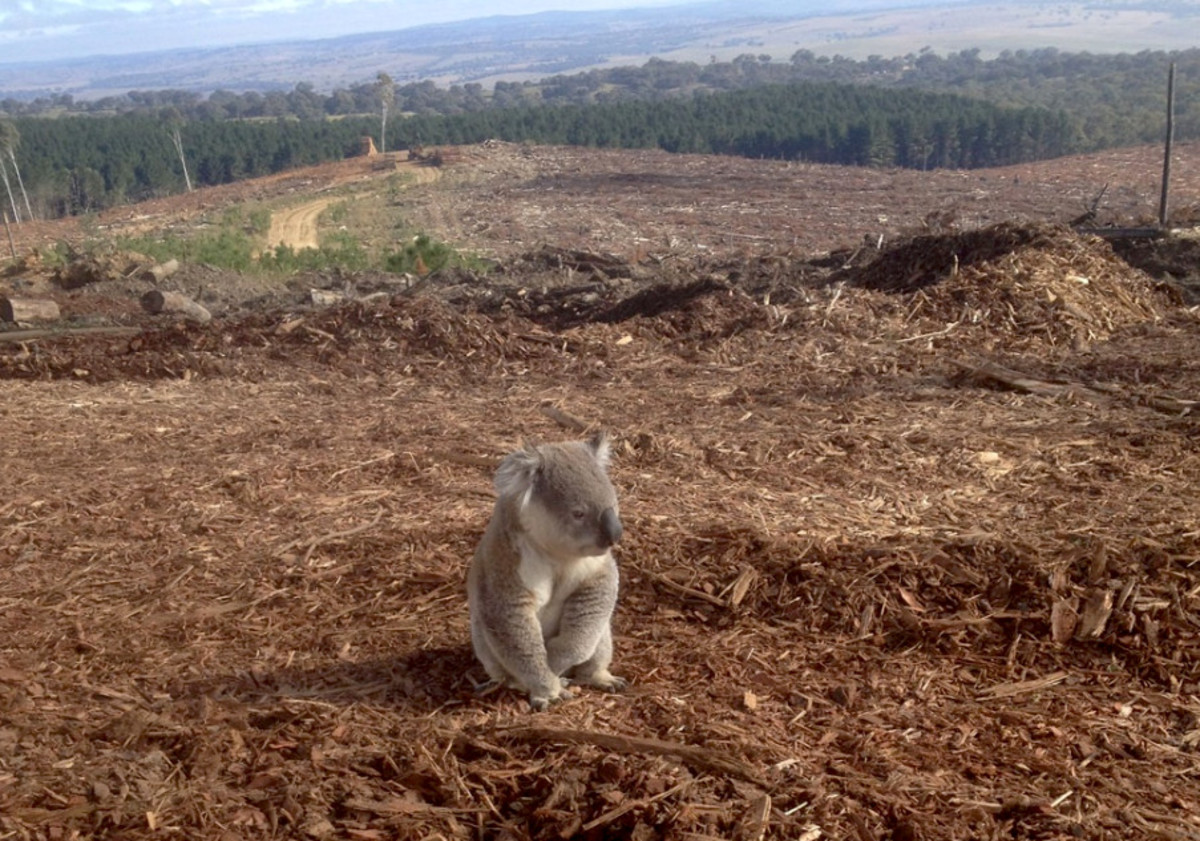In this color photograph, taken in a landscape orientation, the main subject is a small koala bear, situated near the bottom center of the image. The koala, with its short gray fur, creamy white chest, and large brown-gray nose, sits forlornly amidst red-brown woodchips, tree debris, and sawdust, its small rounded ears edged with long fur and paws curled slightly underneath. The setting suggests deforestation, likely in Australia, as there are no trees immediately surrounding the koala, which contributes to its sad demeanor. A gravel path lies to the back left of the scene, while to the back right, the remnants of more chopped trees are visible. A slope behind the koala descends into a large valley filled with green grass and lush, dark green pine trees, creating a stark contrast with the barren foreground. Some skinnier trees, appearing like birch with their white bark and sparse leaves, are visible to the back left, leading into the distant, hazy blue sky. The overall scene evokes a sense of loss and abandonment, highlighting the impact of deforestation.